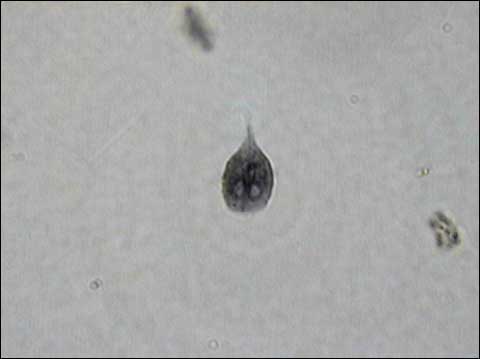The image appears to be a highly magnified view, likely captured via microscope, depicting a central dark gray amoeba or cell with a distinctive rounded body and a pointy tail. The entire image is rendered in black, white, and various shades of gray, contributing to a hazy gray background. The primary focus, the central organism, is set off against this background, emphasizing its dark gray color. Surrounding the main entity, there are a few additional dark gray blobs—one in the top center and another on the middle right—though they are blurred and less defined. The organism itself boasts a pair of black circles with lighter gray centers, resembling eyes. This microscopic scene is enclosed within a thin black trim, and the surface area is dotted with faint gray circles and random deeper gray specks, indicating the presence of other minuscule structures. There is no text in the image, reinforcing the scientific and observational nature of the photograph.